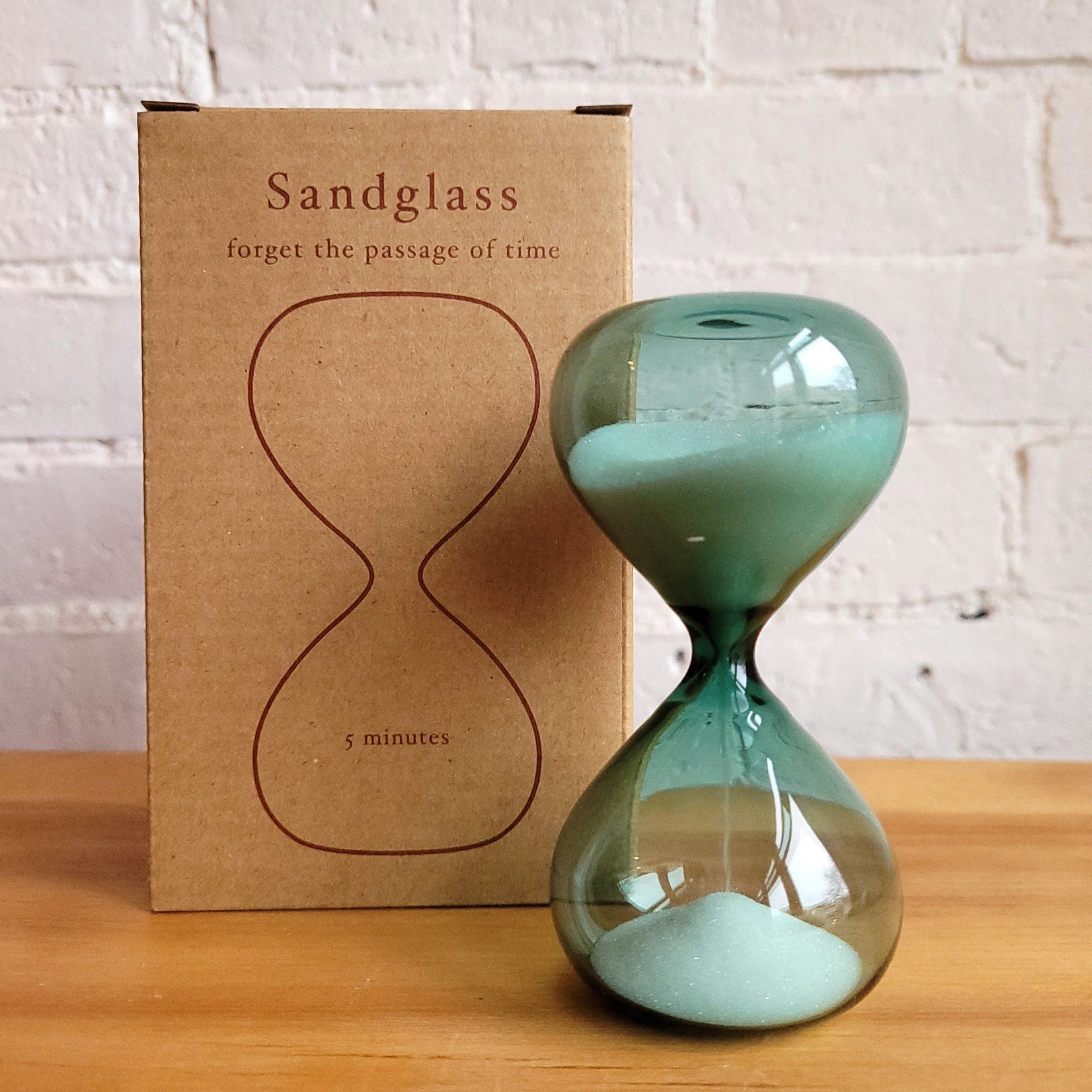This image showcases a turquoise-tinted glass hourglass filled with white sand. The hourglass, capturing time as sand transitions from the top half to the bottom, is situated on a light brown wooden table against a backdrop of a white brick wall. Accompanying the hourglass on the left is its cardboard packaging, a brown box adorned with black lettering. The text on the box reads "sandglass" at the top, followed by the phrase "forget the passage of time," and features a line drawing of an hourglass that denotes a five-minute duration. The hourglass's design features a curvy, slender middle with flat ends, clearly presenting the elegant passage of time as the white sand trickles down.